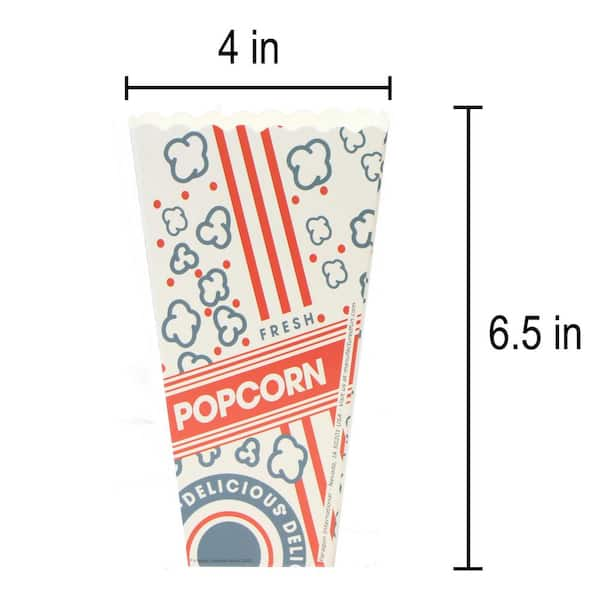This is a detailed, color photograph of a vintage-style, tapered popcorn container, reminiscent of those from the movies. The container is an old-fashioned cup, wider at the top and narrow at the bottom, with a wavy cut edge at its opening. The main design features a white background adorned with scattered images of popcorn outlined in blue, interspersed with red dots. Prominently, three red diagonal stripes extend from the upper left to the lower right.

Across the container's midsection, a bold red band showcases the word "POPCORN" in large white, all-caps letters. Above this band, "FRESH" is inscribed in blue text. Below, a circular label features the word "DELICIOUS" in a repeated pattern. The circle has a blue outer ring and a smaller red circle inside it.

The dimensions of the container are explicitly provided with measuring lines. A horizontal line above the container reads "4 inches" in black text, while a vertical line on the right side states the total height as "6.5 inches." The overall color scheme is subtle, with muted reds, whites, and blues. The image background is plain white, with no popcorn inside the container.